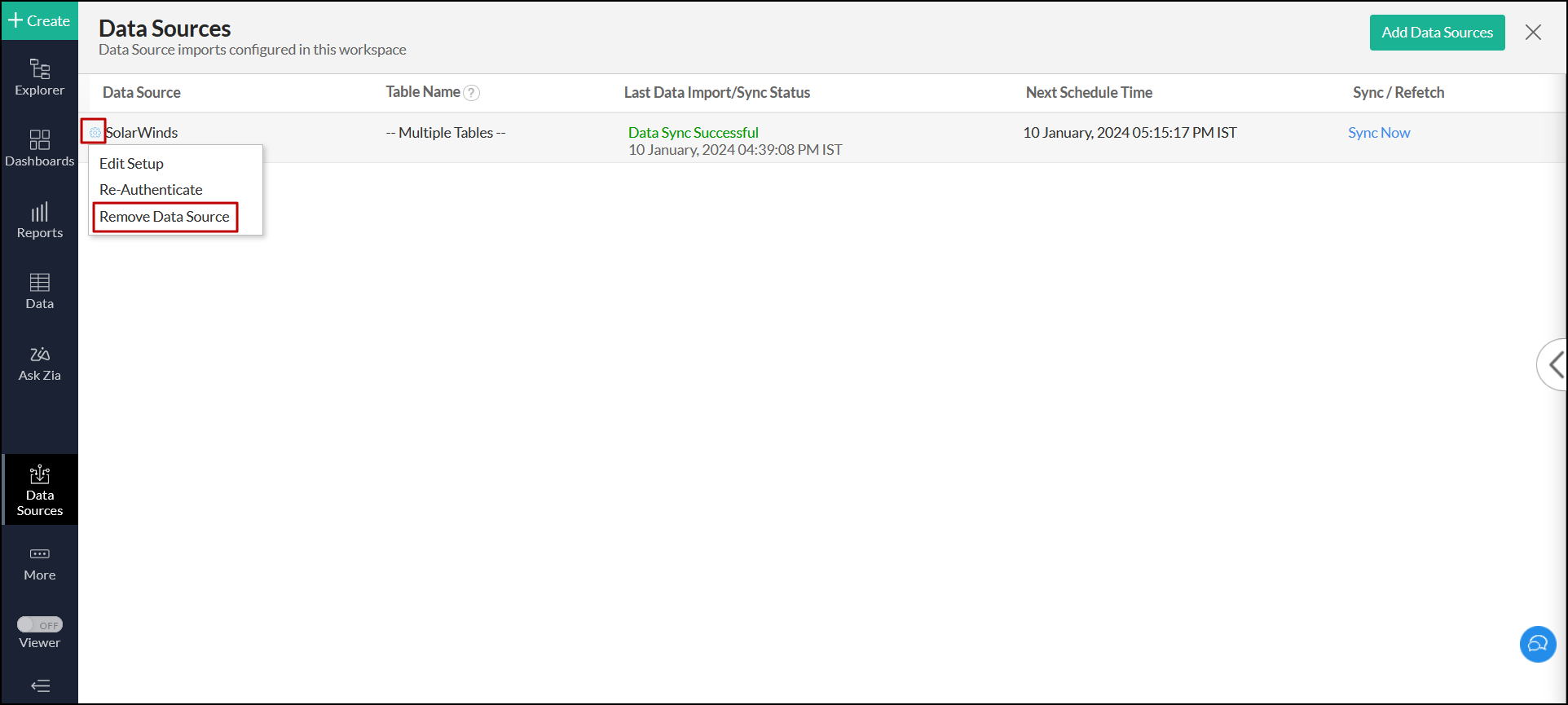A detailed and clean caption for the described image could be:

"Screenshot of a data management interface titled 'Data Sources: Data Source Imports Configured in This Workspace.' The interface displays a table with columns labeled 'Data Source,' 'Table Name,' 'Last Data Import,' 'Sync Status,' 'Next Scheduled Time,' and 'Sync Refresh.'

Underneath the table headings, there is a row for 'Solar Winds.' The row shows 'Multiple Top Tables' under 'Table Name,' 'Data Sync Successful' under 'Sync Status,' and lists the 'Next Scheduled Time' for synchronization as 'January 10, 2024, at 5:17 PM.' A blue 'Sync Now' button is also present in this row.

Options for managing the Solar Winds data source, such as 'Edit,' 'Setup,' 'Authenticate,' and 'Remove Data Source,' are available, with 'Remove Data Source' highlighted in a red box.

On the far left, there are additional options like 'Create,' 'Explore Documents,' and 'Report 11 8A 4S / ID.' Below these, options for 'Some Drop Version' and 'Volume' are also listed."

This caption provides a thorough and detailed description of the visual and textual elements in the screenshot.